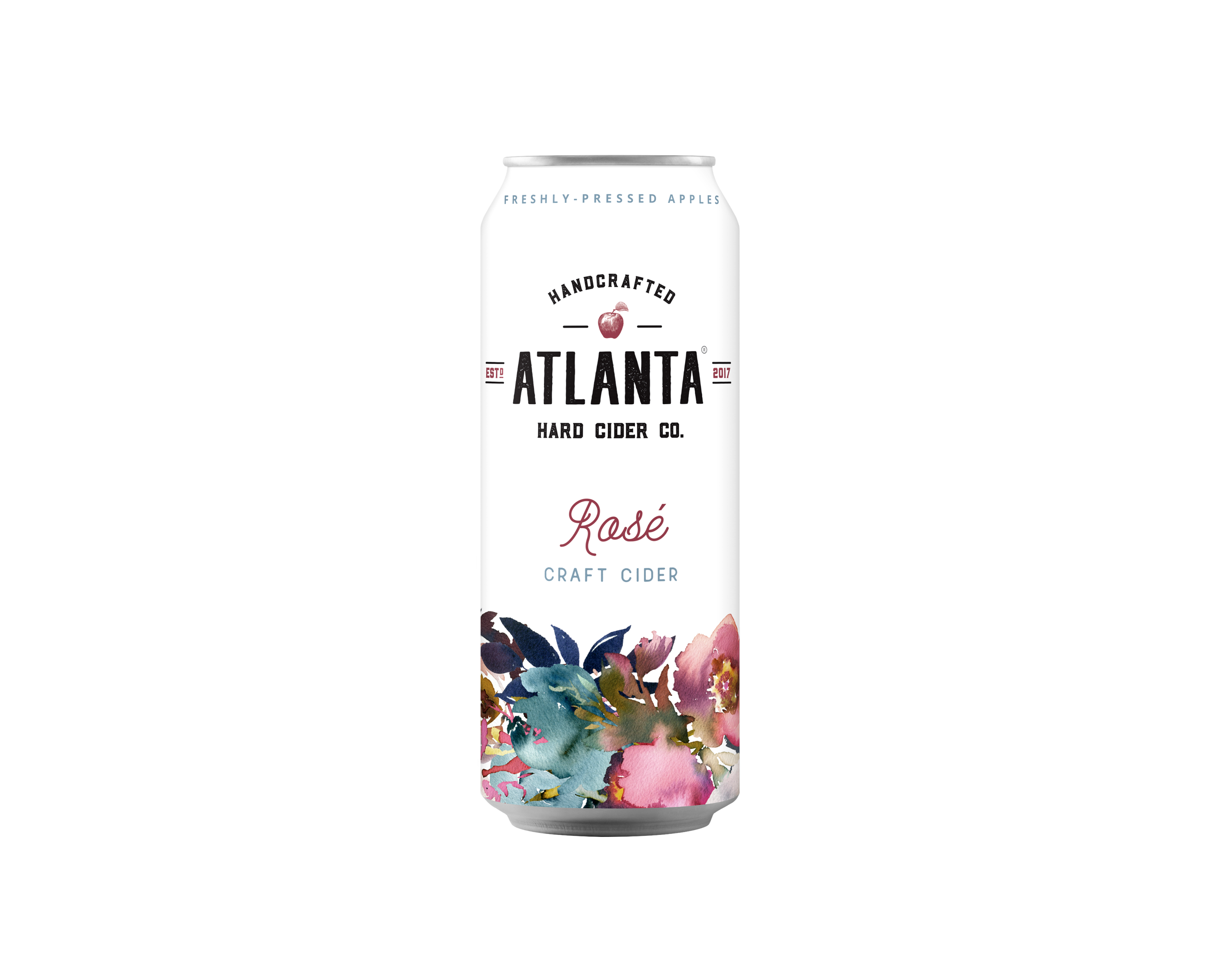The image features a close-up of a tall boy can of handcrafted Atlanta Hard Cider, set against a completely white background. The can itself is primarily white with silver lining visible at the top and bottom. At the top of the can, "freshly pressed apples" is written in gray text. Directly below that, "handcrafted" appears in black text above the logo, which includes a red apple and the words "Atlanta Hard Cider Company" with an "Established 2017" date in red text beside "Atlanta". Below the logo, "Rosé" is elegantly written in red cursive text, followed by "craft cider" in bold, silverish-gray text. The bottom of the can is adorned with an assortment of watercolor-style flowers in teal, dark blue, pink, red, green, and white, adding a touch of vibrant detail to the otherwise minimalist design.